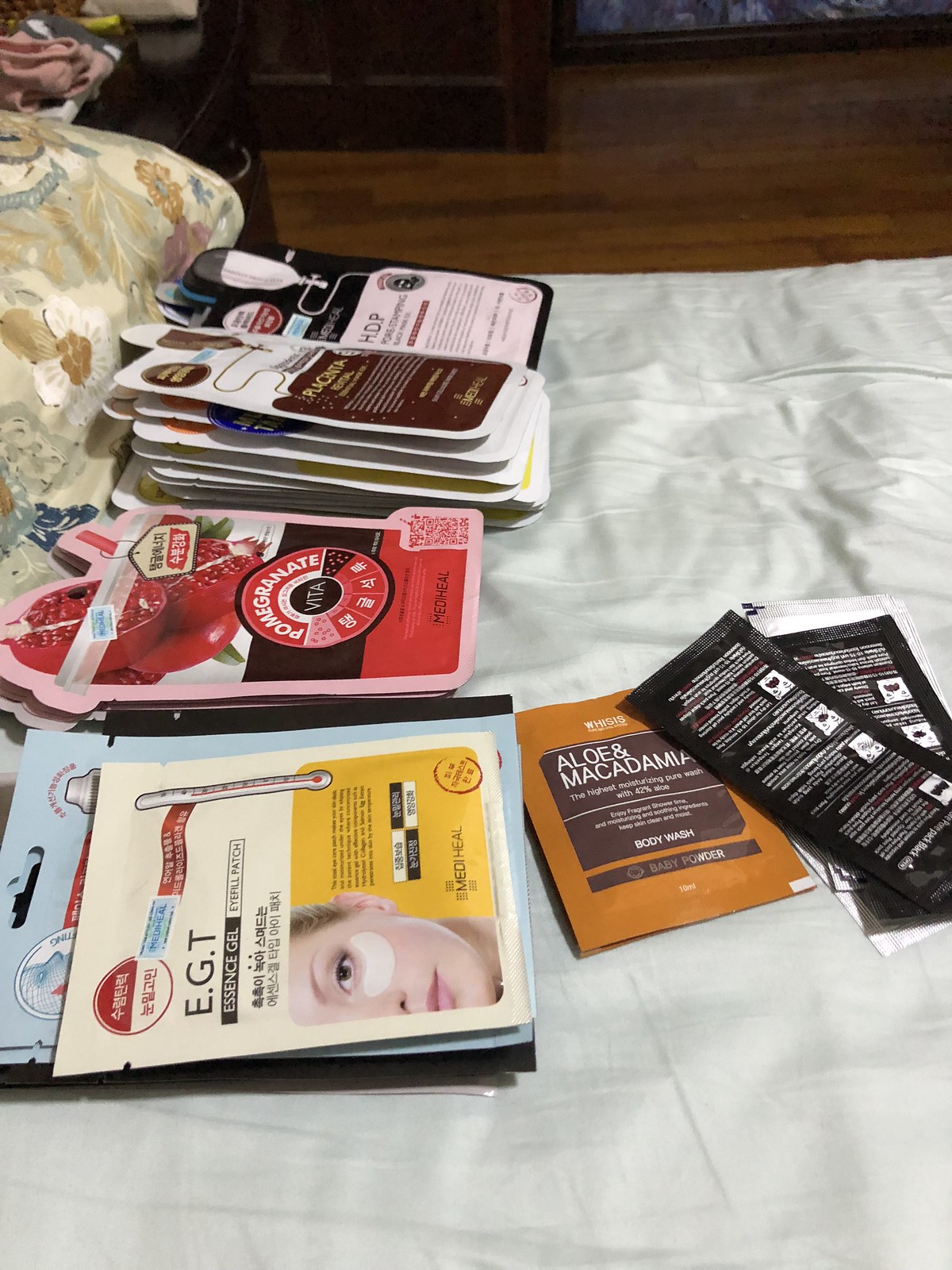A photograph features an assortment of beauty products meticulously arranged on a bed covered with a white sheet. The vibrant collection, constituting four to five distinct stacks, predominantly includes face gels such as EGT Essence Gel, which is applied via patches, as well as a variety of other items like aloe and macadamia body wash, pomegranate treatments, and ADP beauty products. Each stack and packet is neatly organized, creating an aesthetic display of skincare and beauty essentials. The backdrop consists of a colorful pillow adorning the bed and a glimpse of brown wooden flooring and possibly another upholstered seat or couch, adding depth and warmth to the scene.